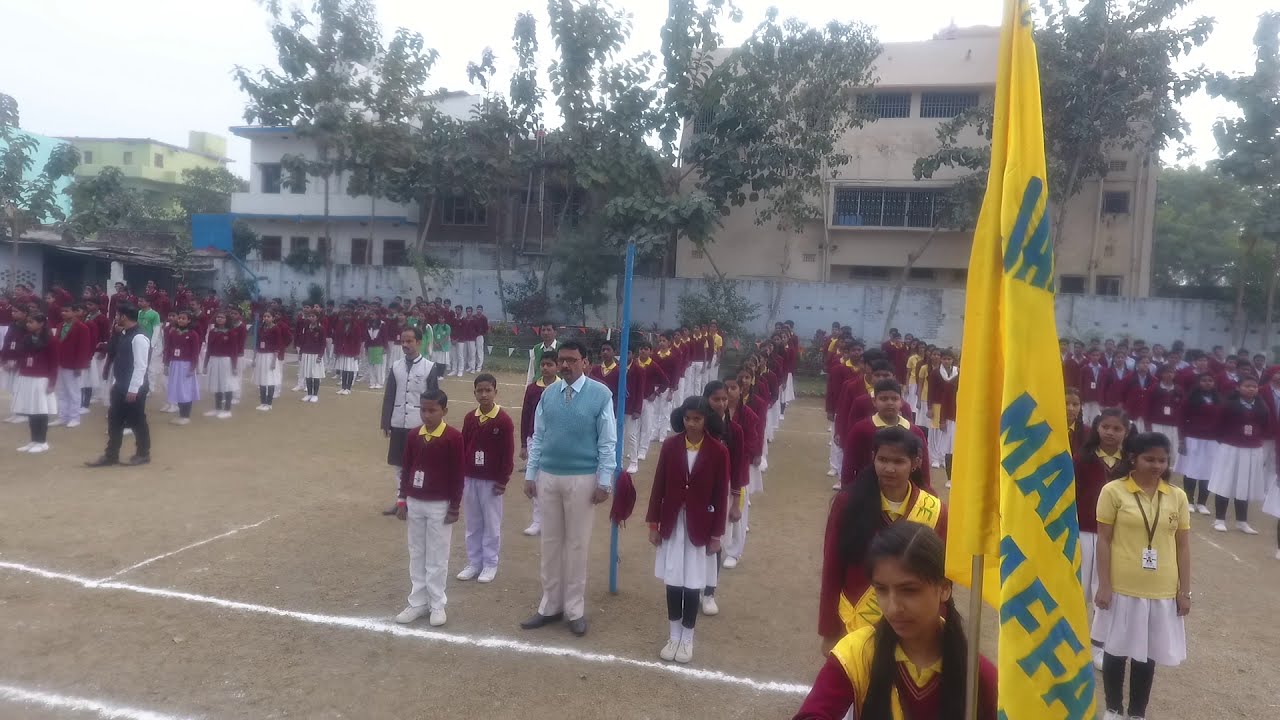The photograph captures a well-organized lineup of students in uniforms, positioned in parallel lines on a brown dirt courtyard with white painted lines. The children, all with dark black hair, are uniformly dressed in red sweaters or jackets. Girls are wearing white skirts, while boys are in white pants. Some students have yellow scarves around their necks or draped over their shoulders, and a girl in the bottom right corner is distinctively dressed in a yellow shirt with a white skirt and a lanyard holding a white ID badge around her neck. 

An adult man, notably taller than the students, stands prominently with a blue shirt beneath a blue vest, tan pants, and dark boots. 

In the background, various buildings in neutral tones of gray, brown, and cream with multiple windows and balconies frame the scene. One building to the right is accented with blue trim. amidst the architectural structures, trees with bright green leaves illuminate the space as sunlight filters through, creating a hazy sky effect. The girl at the front of one of the lines on the right side holds a drooping yellow flag emblazoned with unreadable blue writing.